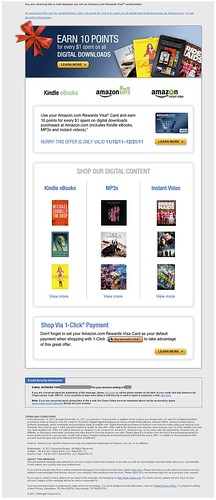The image is a smartphone screenshot showcasing an advertisement for earning points on digital purchases. At the top, a banner promotes the offer: "Earn 10 points for every $1 spent on digital downloads," accompanied by a "Learn More" button. Below the banner, product categories are presented, focusing on various digital content available for purchase. The categories include Kindle eBooks, MP3s, and instant videos, each featuring three thumbnail images of available products. Although the product names are not legible due to blurriness, the sections are clearly delineated. 

Beneath the product display, there's a shopping cart icon and a message urging quick action: "Hurry, this offer is only valid until 11/15/11." Another "Learn More" button is located under this message. Additionally, a separate section near the bottom emphasizes the convenience of shopping via one-click payment, with yet another "Learn More" button for further details. Throughout the screenshot, several "Learn More" buttons appear, encouraging users to explore the offer and the shopping process further.